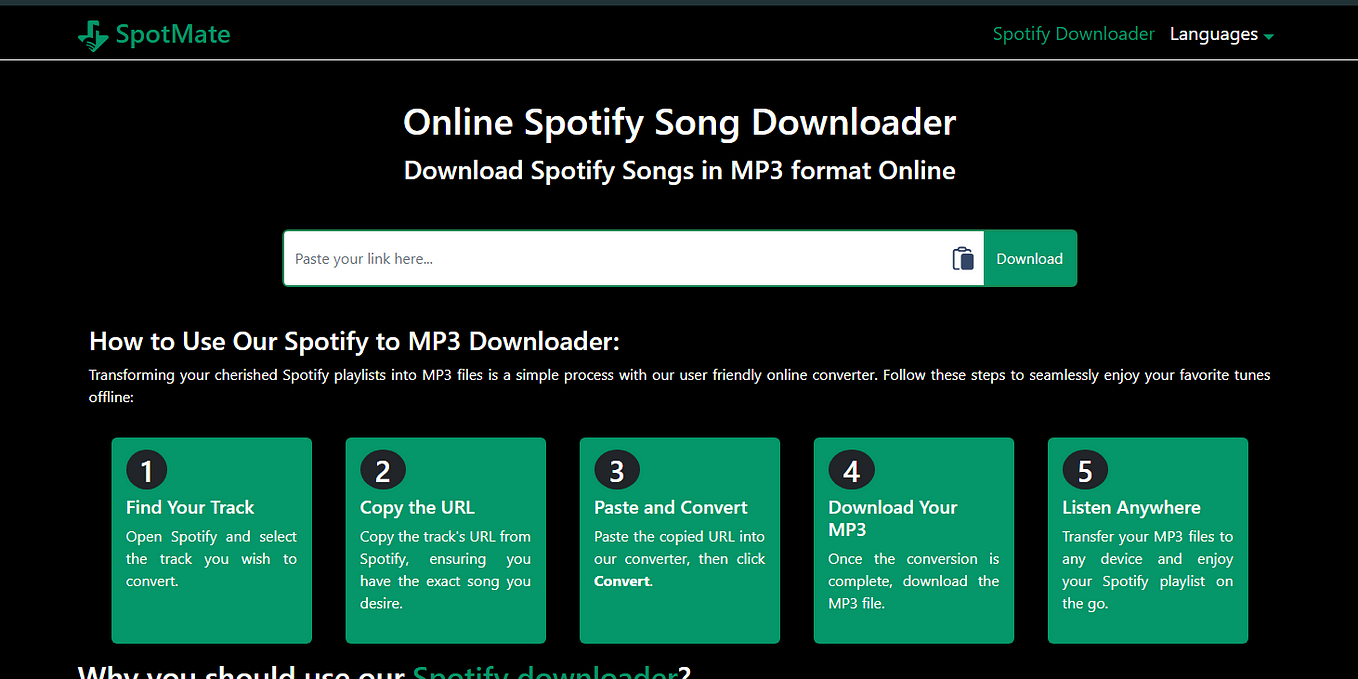The image is a horizontally rectangular screenshot taken from the upper portion of a web page or app, set against a black background. In the top left corner, the text "SpotMate" is displayed in green. On the upper right, "Spotify Downloader" is also highlighted in green, followed by the word "Languages" in white with a green drop-down menu arrow centered beneath this top line. 

Below, a white text reads "Online Spotify Song Downloader" and "Download Spotify songs in mp3 format online." Directly beneath this, there is a text input field labeled "Paste your link here," accompanied by a green download button to its right.

Underneath, there is a section titled "How to use our Spotify to MP3 downloader" in white. It details a simple process for transforming cherished Spotify playlists into MP3 files using their user-friendly online converter. The steps are listed in a horizontal sequence from left to right.

1. **Step 1: Find your track** - A green square contains a black circle in its top left corner with the number "1" inside.
2. **Step 2: Copy the URL** - Similarly, a green square with a black circle containing the number "2".
3. **Step 3: Paste and convert** - A green square with a black circle containing the number "3".
4. **Step 4: Download your MP3** - Another green square with a black circle containing the number "4".
5. **Step 5: Listen anywhere** - The final green square with a black circle containing the number "5".

Overall, the image provides a clear guide on how to use the Spotify to MP3 conversion service, emphasizing its simplicity and ease of use.